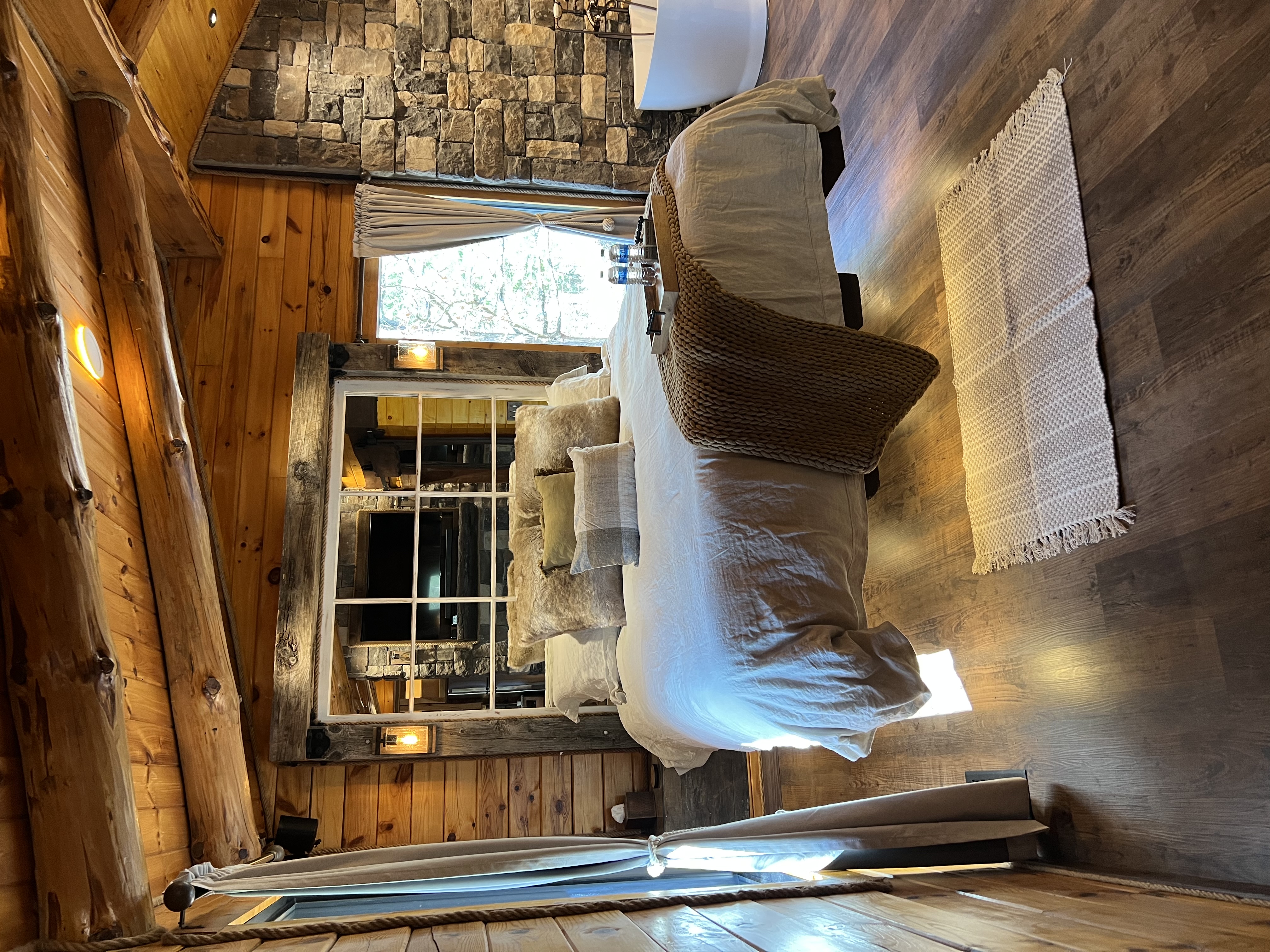This detailed photograph, properly viewed by rotating it clockwise, features a cozy bedroom within a rustic log cabin. The room is adorned with wood paneling on the walls and ceiling, exhibiting exposed log beams that enhance its rustic charm. A low ceiling envelops the space, which includes dark brown hardwood floors and a small, fringed woven area rug at the foot of the bed. The queen-size bed, centrally placed in front of a large window framed by tied-back curtains, is dressed in a tan sheet and a white bedspread, with a brown blanket draped over one corner. The bed is adorned with an impressive array of throw pillows, numbering around seven to nine. At the foot of the bed rests a tray holding two bottles of water, adding a touch of convenience and hospitality to the scene. To the right of the bed, there is a striking gray granite stone wall, partially obscuring a modern white bathtub. Lantern-style sconce reading lights are positioned on either side of the bed for practical lighting. Outside the glass door, a sunny backyard with trees is visible, suggesting a serene and secluded location. The overall ambiance, complete with a cedar log beam visible on the ceiling and recessed lighting, evokes a sense of luxurious yet rustic charm, making it an ideal setting for a vacation rental advertisement in an exclusive mountain cabin retreat.